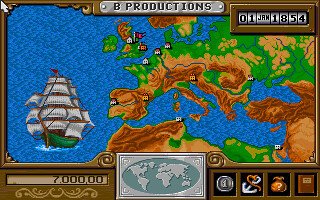The image depicts an antique sailboat navigating calm waters, part of a detailed video game map. The map predominantly features expansive blue waters accompanied by patches of brown, tan, and green landmasses. The title text in the top section reads "B Productions" with a date timestamp of January 1st, 1854, evoking a historical maritime exploration theme.

At the bottom of the image, a figure of "7 million" is displayed, possibly indicating a score, population, or resource count integral to the game's context. Centrally positioned, there is an additional map featuring a silver outer ring, with a green oval interior, and silver landforms within, suggestive of an in-game world or location highlight.

To the right side of the main map, there is a subdivided area consisting of four distinct squares, each containing unique images that likely represent key points of interest or interactive elements within the game. The entire map is framed by an elegant brown trim, providing a classic and cohesive aesthetic to the overall design.